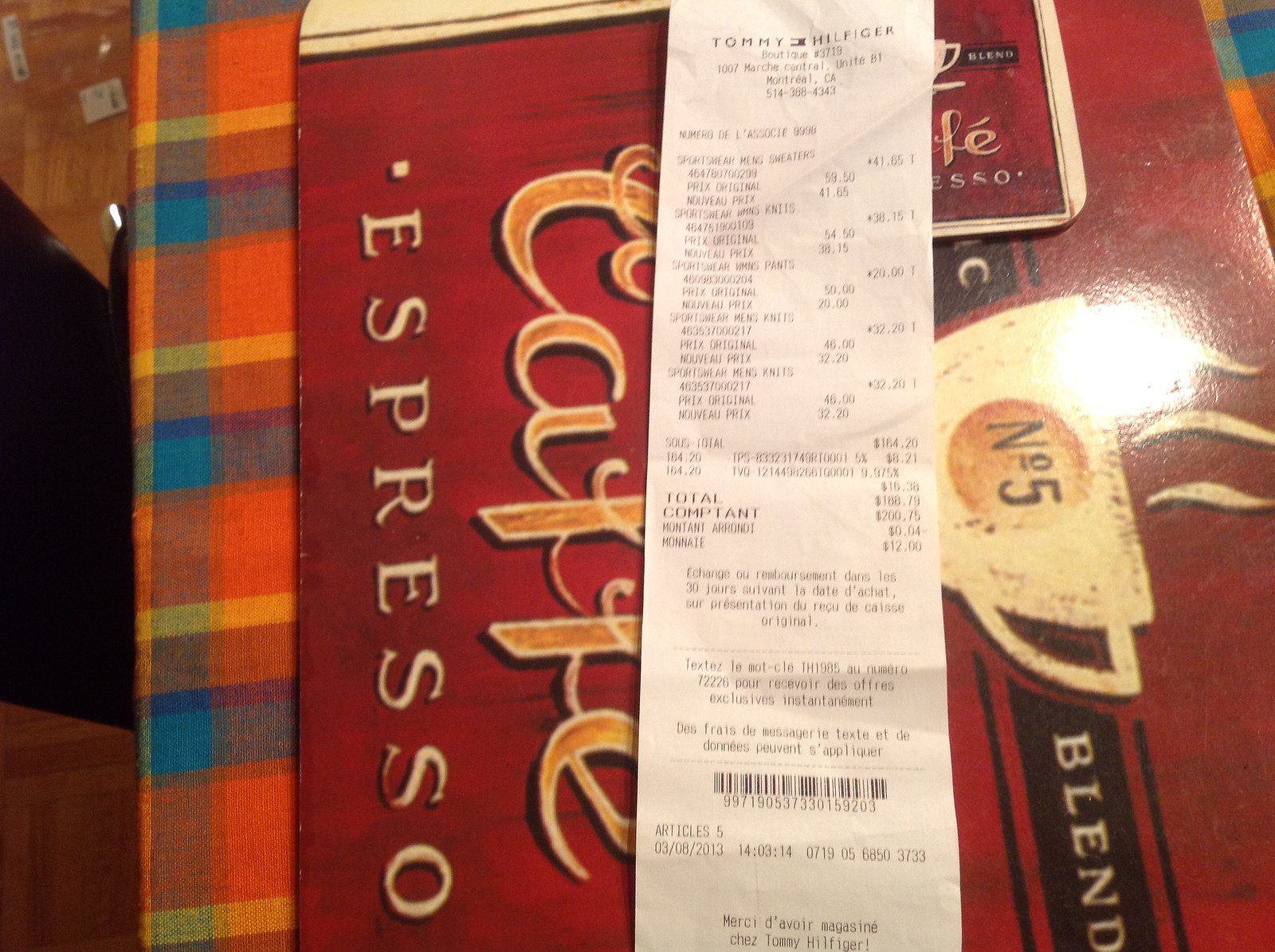The image displays a white receipt from a Tommy Hilfiger store, detailing multiple purchases with prices including $41, $38, $20, and $35, amounting to approximately $200. The receipt, printed in black ink, lists items in both English and some French, and features a barcode and timestamp at the bottom. This receipt is placed on a red, burgundy-toned box, labeled "Caffe Espresso" with various design elements. The box is oriented sideways with black strips bearing white lettering. Prominently, there's an illustration of a white coffee cup with an orange circle and the number "No5" on it, suggesting a blend. Below this, the words "CAFFE" in orange and "Espresso" in yellow run vertically. The box sits on top of a tablecloth featuring a vibrant pattern of blue, yellow, and orange stripes. To the left of the box, a wooden floor peeks into view.